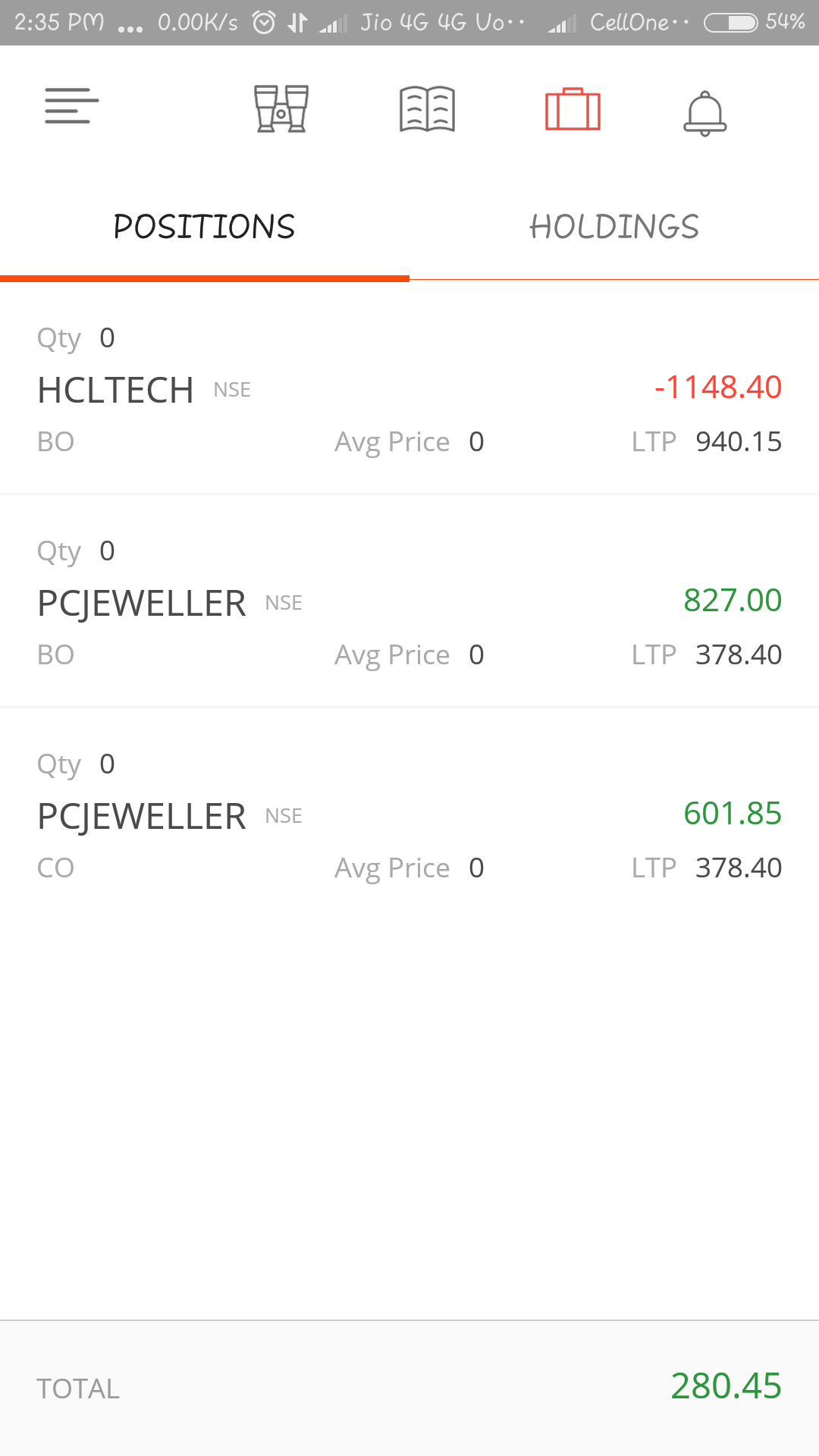**Category: Websites**

**Image Description:**

The image showcases a compact webpage designed for stock tracking, displayed on a mobile phone screen. The phone indicates the current time as 2:35 PM and has an alarm set. At the top of the screen, "Cell 1" is mentioned, and the battery level is at 54%. A menu button is located in the top left corner, along with various icons including binoculars, a book, a suitcase, and a notification bell, presumably for navigation and additional functionalities.

The main content of the page lists stocks being tracked. The first stock is HCL Tech NSE, showing an average price of 0, a negative value, and an LTP (Last Traded Price) of 940.15. Further down, the stock for PC Jeweler is listed with a quantity of 0, a value of 827, and a positive change. The average price remains 0, with an LTP of 378.4. Additionally, there is another entry for PC Jeweler CO, with a value of 60185 and an LTP of 378.40, and totaling to 280.45.

The page is simplistic yet informative, providing key financial metrics and updates in a concise format.